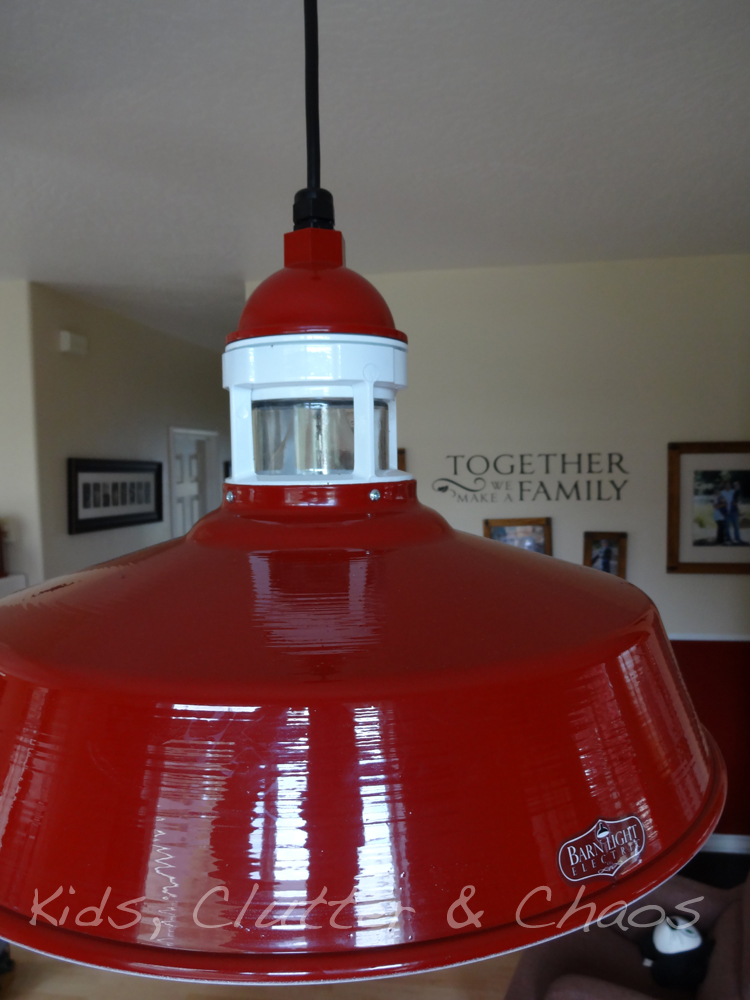The image captures an interior space, possibly a museum, welcome center, or a family home replete with artifacts and informational displays. The soft white walls and ceiling lend the room a clean, welcoming atmosphere, complemented by a white alarm system box stationed high on one of the walls. A cozy ambiance is supported by a tan wall and various family photographs framed in subdued brown hues and arranged neatly across the backdrop. A prominent photo emblazoned on the wall bears the heartfelt inscription, "Together, we make a family."

The focal point of the image is an unusual and striking red and white object situated centrally in the room. This object, possibly art or a decorative piece, resembles an oversized, upturned bowl or perhaps even an abstract representation of a lighthouse. The object has a glossy red finish with a narrow white cylindrical section at the top, featuring small windows and capped with a white dome, from which protrudes a slender black rod.

An inscription on the object reads "Barn Light Electric," indicating its possible origin or brand. Additionally, the image contains an overlaid text in a translucent, italic font that spells out "kids, clutter, and chaos," further characterizing the ambient environment as one filled with familial warmth and organized commotion. The room also includes a white door and a horizontally stretched frame containing multiple smaller images, adding to the sense of a lived-in, well-loved space.